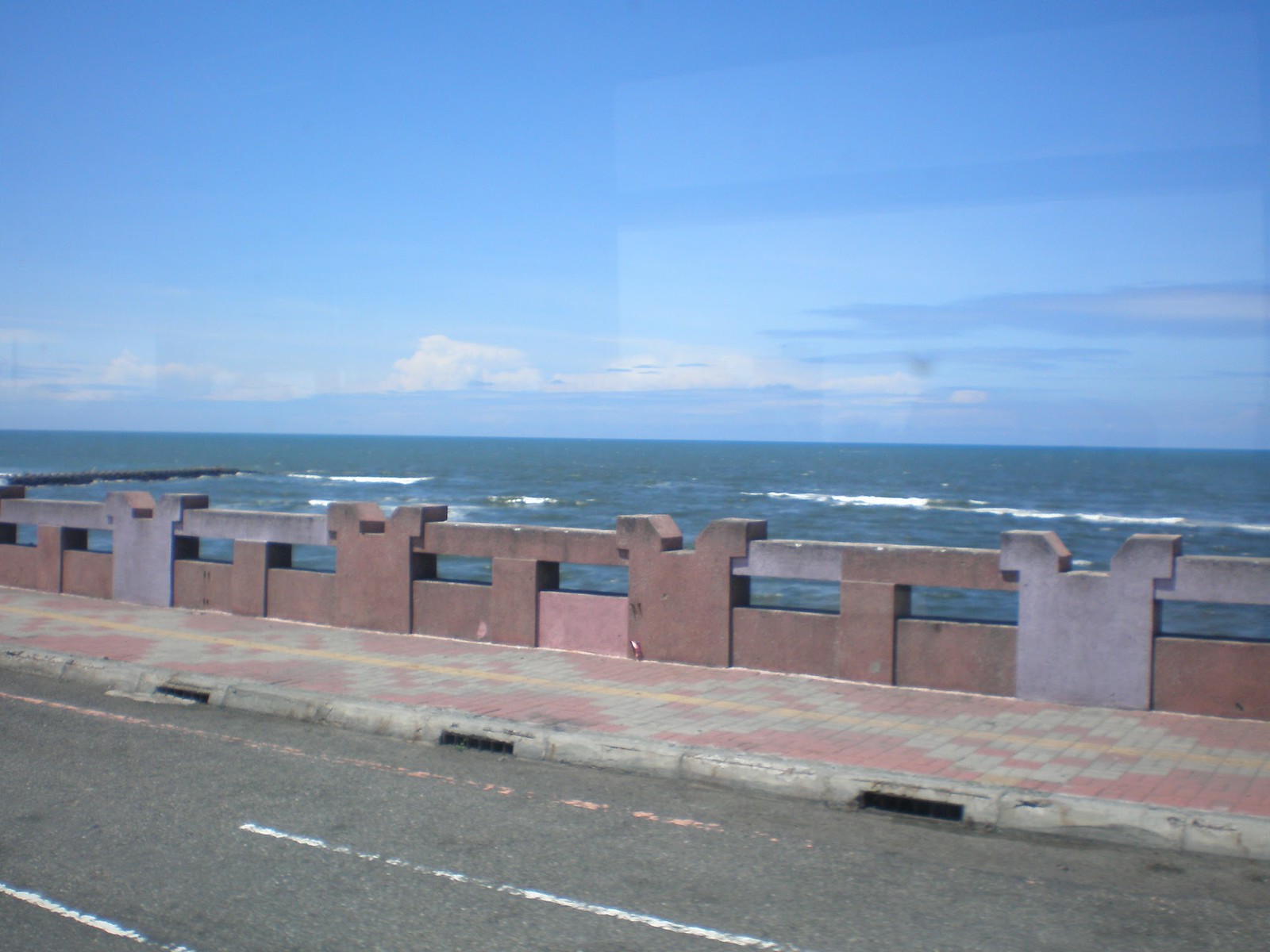This outdoor photograph presents a scenic ocean view from a roadside vantage point. Dominating the foreground is a paved asphalt road, adorned with white stripes and a distinct solid pink line, running diagonally from the bottom right to the middle left of the image. Adjacent to the road is a sidewalk featuring an intricate, symmetrical pattern composed of gray, red, yellow, and green bricks, with three drainage slots visible. A yellow line runs down the center of the sidewalk, which is bordered by a multicolored stone railing—showcasing hues of red, white, pink, and gray— separating the pedestrian path from the expansive blue ocean. The tranquil sea, exhibiting small waves, extends into the distance under a clear blue sky scattered with white clouds. A notable feature in the middle-left of the image is a pier jutting out into the water, adding to the serene coastal atmosphere.